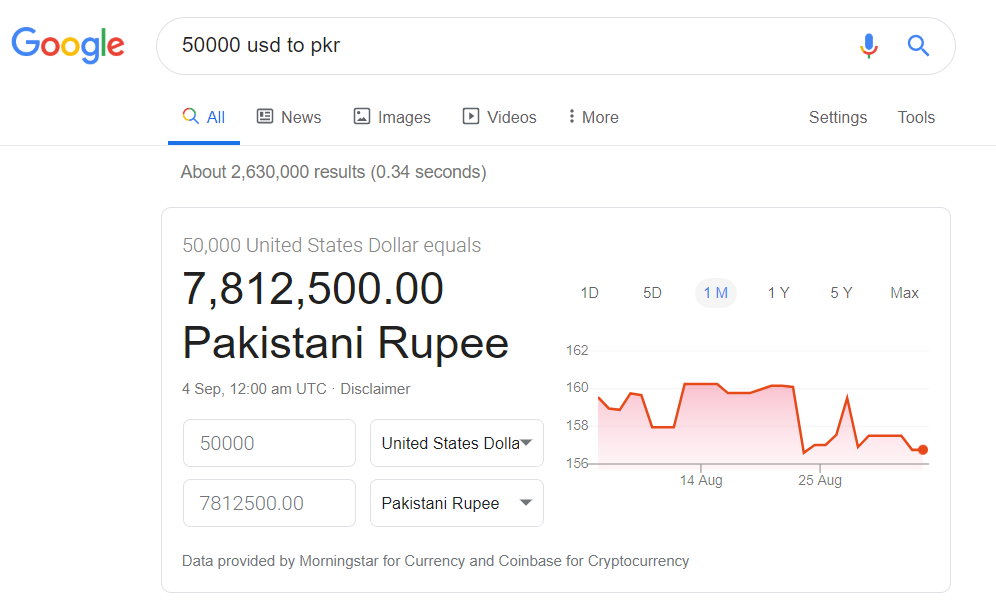The image showcases a Google search result for "50,000 USD to PKR" on a white background. At the top, there's a microphone icon for voice search, followed by a magnifying glass symbolizing the search button. The search terms are underlined in blue, with options to view "All," "News," "Images," and "Videos," alongside three vertical dots for more settings and tools.

The search yields approximately 2,630,000 results in 0.34 seconds, as indicated in parentheses. The conversion displayed shows that 50,000 United States Dollars (USD) is equivalent to 7,812,500 Pakistani Rupees (PKR) as of September 4th, 12:00 AM UTC. Below this, there's a disclaimer followed by a note that the data is provided by Morningstar for currencies and Coinbase for cryptocurrencies.

A graph is also present, displaying various time frames of currency value (1D, 5D, 1M, 1Y, 5Y, and max) with the "1M" (one-month) option highlighted in gray. This graph is positioned at the bottom, offering a visual representation of the exchange rate fluctuations.